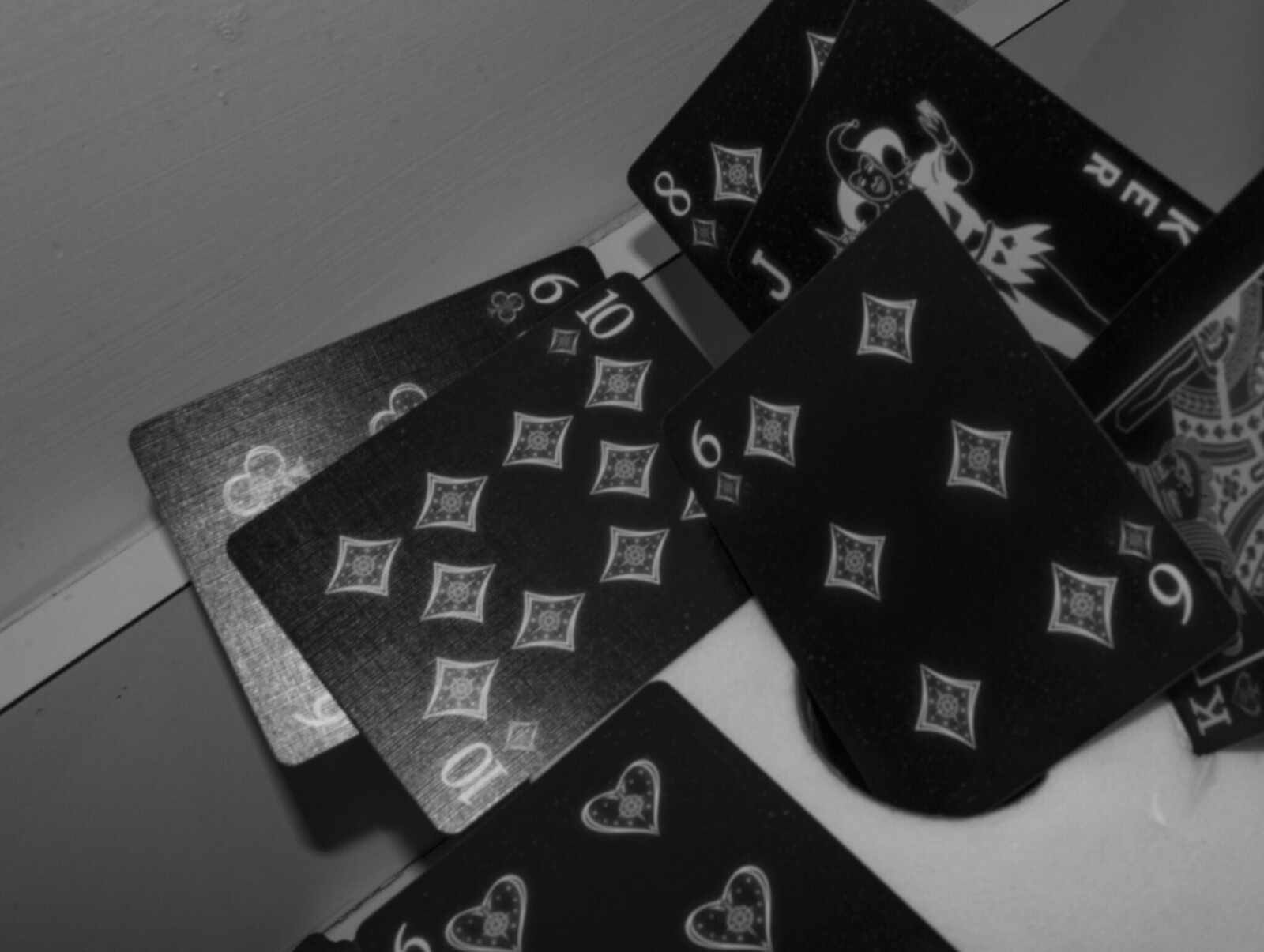The image in black and white captures an intriguing scene within a building, framed by its imperfectly painted wall visible at the top left. Horizontal creases scar the wall's surface, suggesting a hasty or aged paint job. The bottom portion of the image is strewn with playing cards, creating a chaotic yet fascinating tableau. 

Starting at the bottom left, an upside-down card with a pure black back lies inconspicuously. Adjacent to it, there's a card featuring what appears to be the six of hearts, partially showing the heart symbols at the top left, top right, and middle right. Rising slightly above this six of hearts, centrally located in the image, is the ten of diamonds, proudly displaying its number in white text alongside ten diamond shapes.

To the left of the ten, the far-left bottom edge of the six of spades peeks out, teasing viewers with just a glimpse of its spade symbols. In the top right section of the image, a joker card is visibly turned on its side, oriented to face the viewer. The joker's depiction is complemented by the letter "J" at the card's top left corner. Finally, off to the far right, an inverted king card displays the regal figure of a king, adding to the intriguing spread of cards.